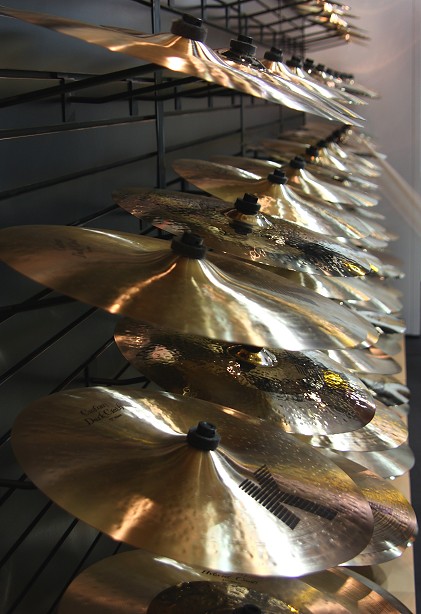This indoor color photograph captures a close-up view of a wall-mounted display of numerous musical cymbals in a music store. The focal point is a black side wall equipped with black racks that elegantly showcase the cymbals, neatly arranged in four horizontal rows with approximately ten cymbals in each row. The cymbals, varying slightly in size, share a uniform shiny gold color, with some reflecting the light, creating striking highlights that resemble white stripes. At the forefront, one cymbal prominently features a large black "K" logo. The cymbals exhibit different textures, with some being smooth and others dimpled. Although slightly out of focus, the composition draws attention to the polished surfaces of the cymbals, contrasting against the plain backdrop of an off-white wall.